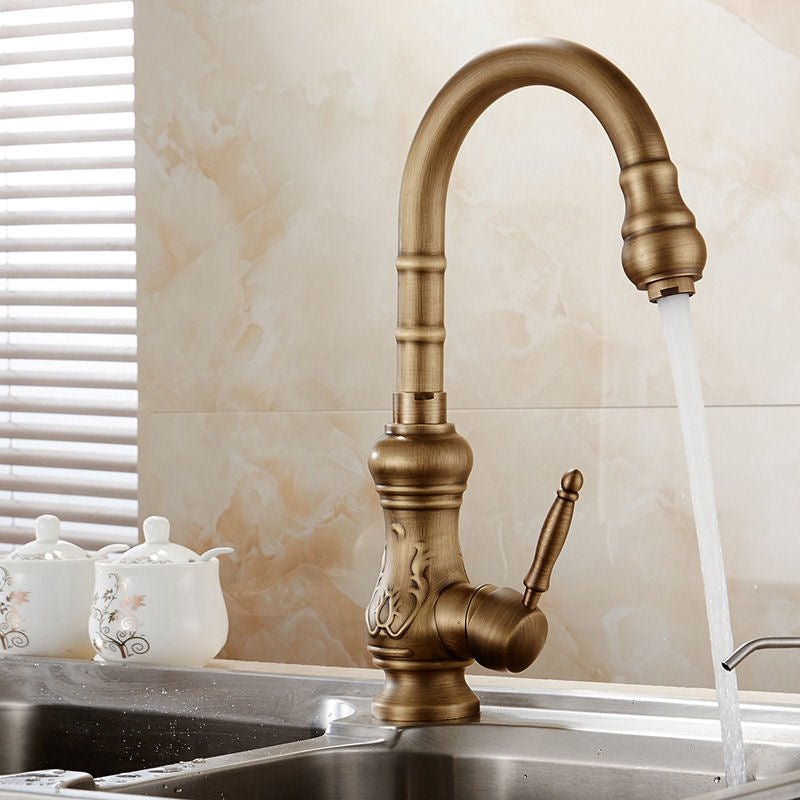This detailed photographic image, set indoors, captures the central focus of a bronze-colored, ornately designed kitchen faucet turned on, releasing a vigorous stream of water into a double-compartment stainless steel sink. The faucet, featuring a single, graceful stem handle adorned with a knob, has a curved neck with two decorative bands and culminates in a U-shaped spout. Water droplets are visible in the air near the left basin, underneath a backsplash of large, creamy white tiles with a subtle marbled tan and beige design. To the faucet’s left, situated in front of a partially visible horizontal mini blind-covered window, sit two white china creamers or sugar bowls with tree and pink flower decorations. On the right side of the faucet, hinting at the image's edge, is the spout of a liquid soap dispenser. The entire scene emanates a rich, detailed realism, from the intricate faucet and droplets of water to the ambient, warm kitchen setting.